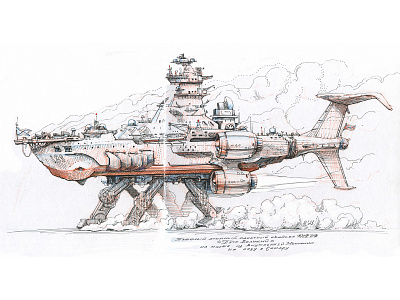This detailed sketch portrays a whimsical, multi-faceted machine that seems to be a hybrid between a boat, submarine, and airplane, with a distinctly mechanical and slightly fantastical twist, reminiscent of something from Star Wars. The machine features a boat-like body and a submarine-like top, with the tail resembling an airplane’s stabilizer. It stands on four brown, articulated legs, giving it a walking appearance, as if it's marching on water. The sketch is colored in shades of pink, with lighter pink and white highlights, accentuating its three-dimensional form. Surrounding the machine are numerous clouds and smoke, adding to the dynamism of the scene. The background is primarily white and gray, enhancing the contrast and emphasizing the detailed artwork. There are also propellers visible on the sides of the machine, and it has multiple levels in the midsection, resembling a tower. Below the drawing, several lines of black text are present, but they are too blurry to decipher. The entire scene has a cartoonish, almost robotic aesthetic, further providing a playful and imaginative interpretation of what seems to be a walking ship navigating through its environment.